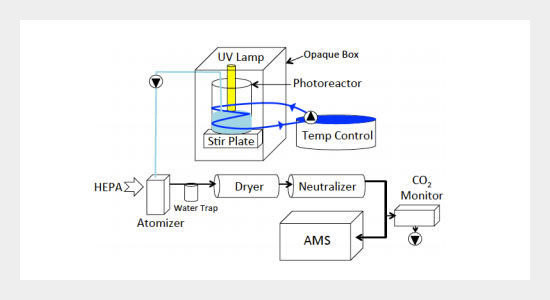The image is a mock-up of an organizational chart for a dryer system, primarily illustrated in black and white with some colored elements. At the top, a cube labeled "UV Lamp" contains a beaker with a yellow tube passing through it, sitting on a stir plate with blue liquid inside. This setup, referred to as an "Opaque Box" and a "Photoreactor," is connected to a "Temp Control" via a blue arrow. From the left of the UV Lamp cube, a tube extends down to a rectangle labeled "HEPA," which links to an "Atomizer." This atomizer directs flow to a cylindrical "Water Trap," followed by another cylinder labeled "Dryer." The sequence continues to a similarly shaped "Neutralizer," with an arrow branching off midway that guides the flow through an "AMS" and a "CO2 Monitor," which is denoted as a smaller rectangular box with a circular arrow. The detailed diagram uses boxes and cylinders to represent different components and colored arrows to indicate flow direction and control points.